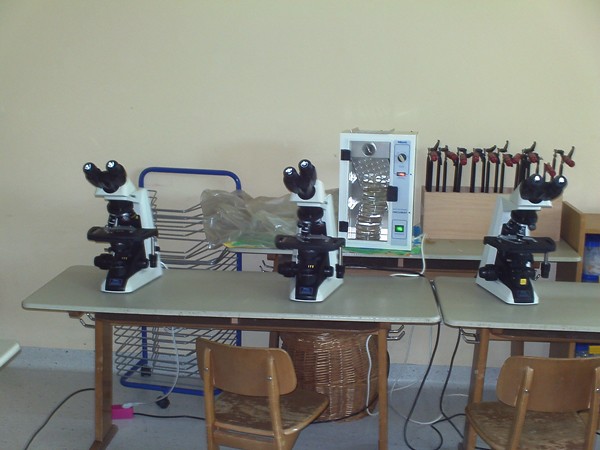The image depicts a modern classroom or laboratory setting equipped with three contemporary microscopes, each black and white in color. The room features two brown chairs paired with tables that have gray tops and brown support structures. The tables are arranged with two in the foreground and one against a light green wall in the background. The tables are neat and modern, one holding two microscopes while the other has one. Underneath the tables, power cords for the microscopes are visible, as well as a brown basket. 

At the back of the room, there is an enigmatic piece of lab equipment with metal components and dials, possibly a heating element. To the left, there is a blue file stand with silver horizontal bars for organizing files. Additionally, a wooden box containing brown sticks and other materials rests on one of the tables. Various objects, including some plastic items and wires, are scattered on the table surfaces, and a blue wired rack is positioned in the back corner, adding to the organized chaos of a functioning educational or research space.